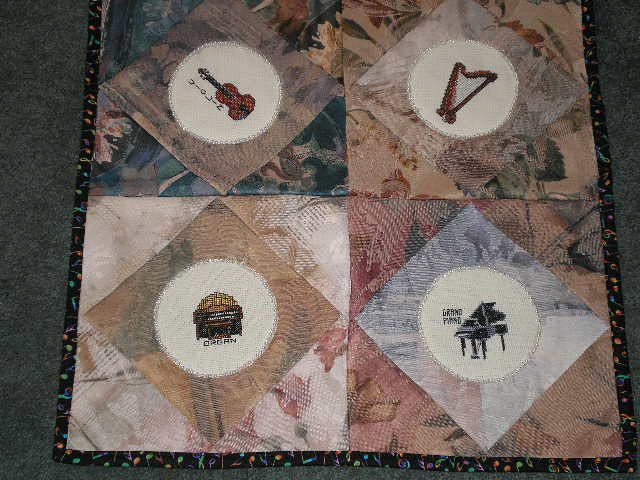The photograph depicts a detailed quilt, potentially a rug, laid out on a fur-like or carpeted floor. This quilt is characterized by its division into four distinct square sections. Each section contains a central diamond made of a rotated square, within which a circular design frames a cross-stitched musical instrument. The instruments showcased include a violin in the top left, a harp in the top right, an organ in the bottom left, and a grand piano in the bottom right. Surrounding these diamond designs are various floral patterns, including tulips and other flowers. Additionally, the perimeter of the quilt features a black trim adorned with colorful musical symbols, including staffs, single notes, and treble clefs. The intricate patchwork and cross-stitching techniques highlight the quilt's artistic craftsmanship and musical theme.